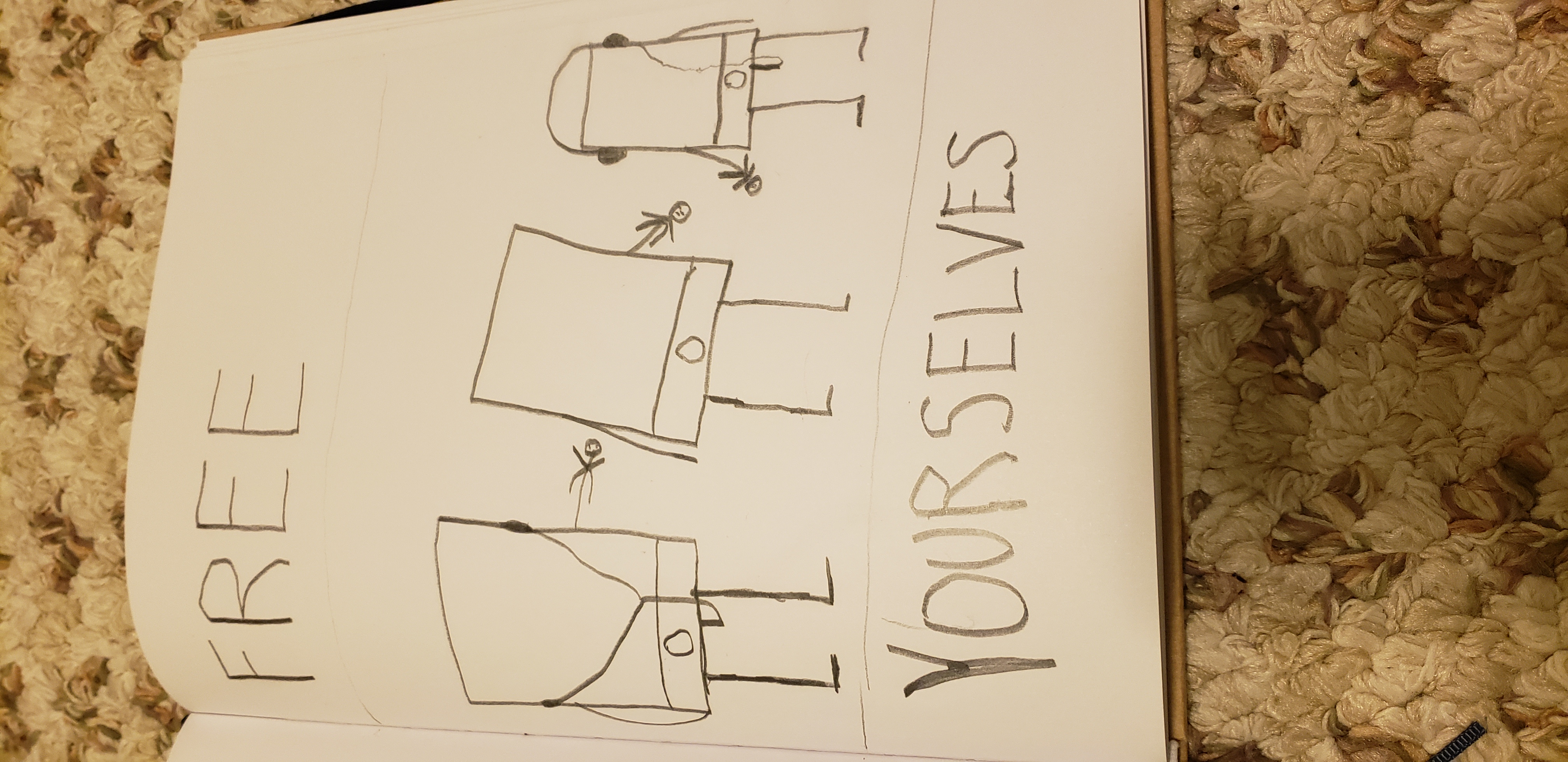This is a color photograph of a page from a sketchbook, oriented sideways. At the very top of the page, written in all capital letters, is the word "FREE." Similarly, at the bottom of the page, also in capital letters, it says "YOURSELVES." Between these two phrases, there are three schematic drawings depicting stick figures. Instead of heads, these stick figures have squares, which resemble either smartphones or television sets. The squares, each with two stick legs, seem to symbolize the restrictive influence of technology on individuals.